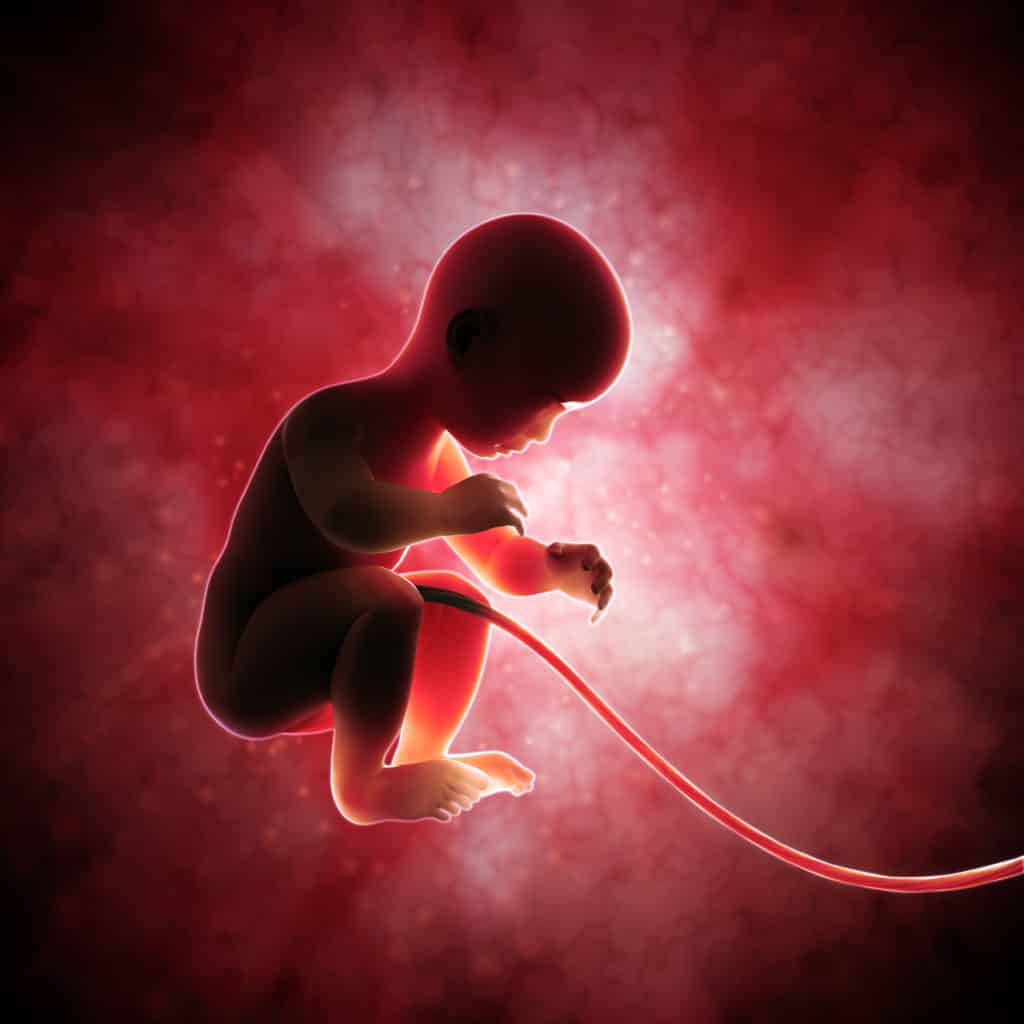This image captures a nearly fully-developed baby in a fetus form, suspended and connected by a long, red umbilical cord that extends off-screen. The baby, facing towards the right with knees curled up to its chest, appears to be floating in an ethereal, womb-like environment. Its flesh-toned skin glows subtly red in areas where light penetrates through, particularly the translucent parts of its feet and left leg, which enhance the ethereal effect. The background is a dark gradient that transitions from black at the edges to vibrant hues of red, pink, and ultimately a bright, glowing white at the core. Intricate red squiggly lines are scattered throughout this gradient, adding texture and depth. The brilliant, almost sunburst-like light at the image’s center illuminates the baby from behind, creating a striking, luminous outline around its form which contrasts with the darker, shadowed silhouette of the baby itself. This radiant lighting accentuates the baby’s features, including its head, ears, fingers, and toes, illustrating its near readiness to be born.